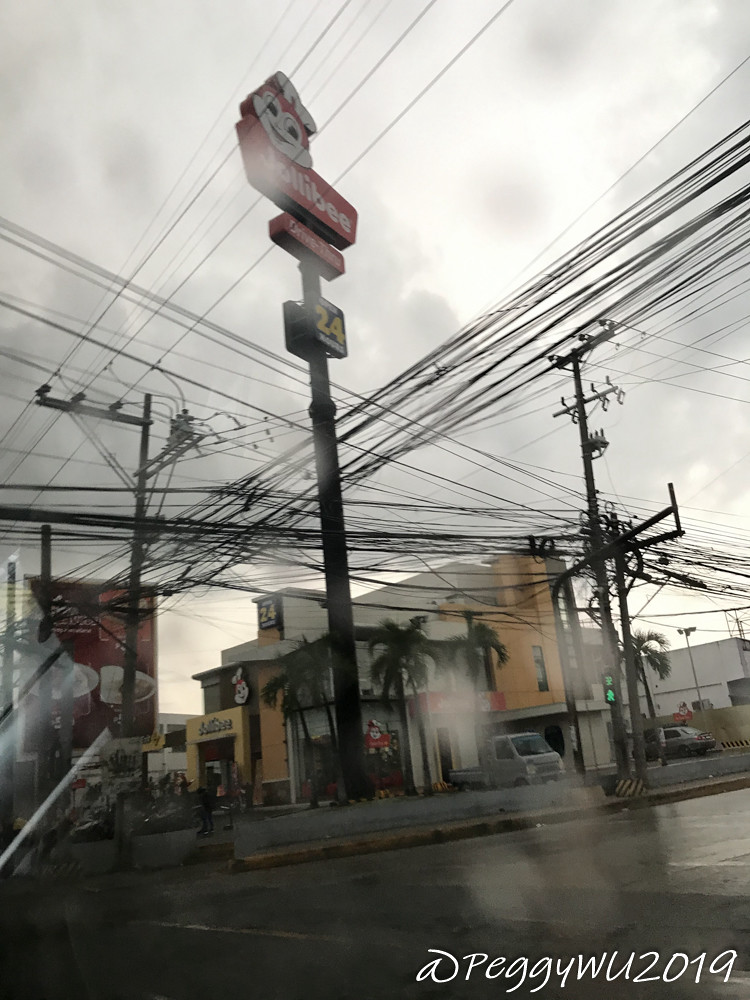The photograph, captioned "At Peggy Wu 2019," captures an outdoor, cloudy scene, possibly during a rainy day, as evident from the blurring caused by raindrops on the camera. The image is primarily of a Jollibee fast food restaurant, renowned for its Filipino menu items like fried chicken and sweet spaghetti, potentially taken from across the street. The Jollibee store building, with distinctive colors of yellow, white, and red, is set against a dark, stormy sky filled with dark gray clouds. The Jollibee sign, indicating 24-hour service, stands prominently from the ground up. The building, which features palm trees at each corner, has a couple of trucks parked nearby. The scene is crisscrossed with numerous intersecting power lines running left to right and at 90-degree angles, adding a sense of complexity to the dreary, rain-soaked atmosphere.